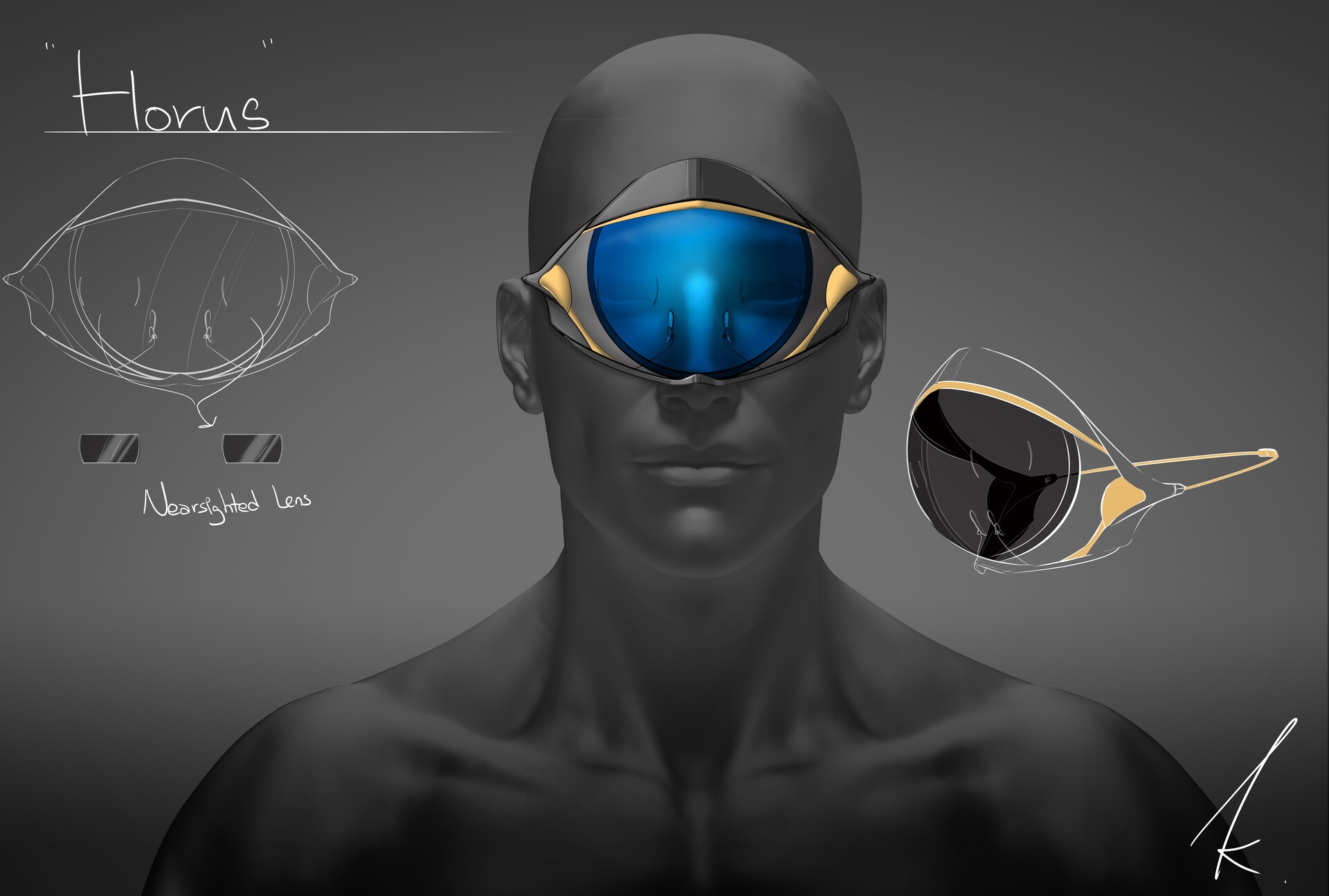The image features a predominantly black and dark gray background. Positioned centrally is a computer-generated, hairless figure with grayish-black skin. The person, whose gender is indeterminate, is wearing a unique pair of virtual reality goggles characterized by a large, eye-shaped blue lens at the center, with gray straps extending to the ears and a yellow section running from the temple to the nose. 

To the right of this figure is a side sketch of the goggles depicted in black. In the top left corner of the image, "Horus" is written in capitalized white letters above a small white sketch that resembles a jellyfish. Directly beneath this sketch are two rectangular black bars with gray stripes, followed by the caption "Nearsighted Lens." In the bottom right corner of the image, there is a large white letter 'K.'